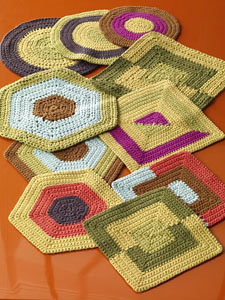This is a small color photograph depicting a collection of crocheted hot pads and coasters in various colors and shapes, neatly arranged on a light orange surface, likely a table. The patches are interlocked and overlapping, consisting of squares, circles, and hexagons with distinct, almost symmetrical geometric patterns. Each patch incorporates different colors, including shades of purple, red, brown, blue, white, and notably, a recurring buttercup yellow. Made from a fuzzy material, the patches exhibit a hand-crafted charm, with intricate designs that differ from one another yet maintain a cohesive visual harmony. For instance, the patch in the lower right-hand corner features a light yellow and khaki green geometric design, while the adjacent hexagonal patch boasts a blue center, a pink outer ring, and a yellow rim.